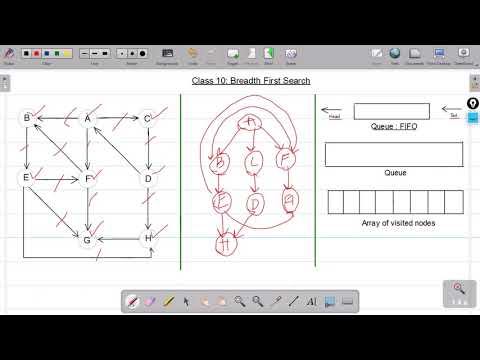The image is a pixelated screenshot of a digital rendering created in a software application, possibly a Microsoft program, featuring a variety of creative and graphical tools. The interface shows upper and lower gray toolbars containing icons such as an eyedropper, magnifying glasses, an eraser, and paintbrushes, allowing the user to select colors and utensils for drawing.

At the center of the canvas is prominently displayed text reading "Class 10: Breadth First Search," which is underlined. On the left side, there is a hand-drawn flowchart in a vertical rectangular layout. This chart consists of various points labeled with letters A through H, connected by arrows in different directions, including some surprising sequences like B to E, E to F, F to B, D to A, C to D, and E to G. The arrows link these letters in a mix of straight and diagonal paths, forming a complex web of connections. Some arrows and letters are highlighted with crosshatches or red check marks, possibly corrections made by an instructor.

In the middle of the canvas, a second hand-drawn flowchart presents a different arrangement of the same letters, this time encircled in red with arrows connecting them in swirling, circular patterns.

On the right side of the canvas, three blank form fields are depicted. The top form field is labeled "Q FIFO" with an empty square above it, the second is a rectangular field labeled with text that is difficult to read due to compression, and the third field consists of gridded squares labeled "Array of Visited Nodes."

Overall, the image combines graphical representations and form fields to illustrate the concept of breadth-first search, enriched with visual aids and corrections, indicative of an educational or research setting.